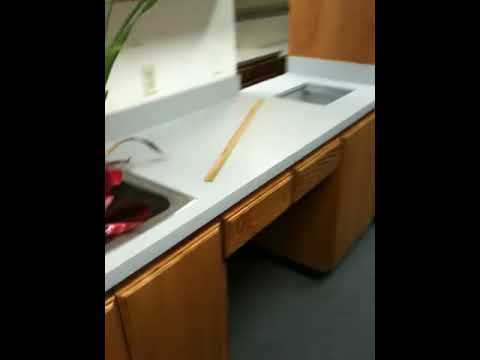The image depicts an indoor scene with low lighting, imparting a grainy texture to the photo. It has vertical black borders on the left and right sides, but no borders on the top and bottom. The central focus of the image is a gray kitchen countertop, angled slightly, creating a downward slope from the upper right to the lower left corner. Positioned diagonally across the countertop is a wooden yardstick with black print, exhibiting a darker yellow hue. The countertop is against a beige or pale white wall, which features an off-white receptacle outlet and a white receptacle cover without any outlets to the right of it. The backsplash on the counter aligns with the wall, and beneath the counter are two wooden drawers, notable for their lack of visible handles.